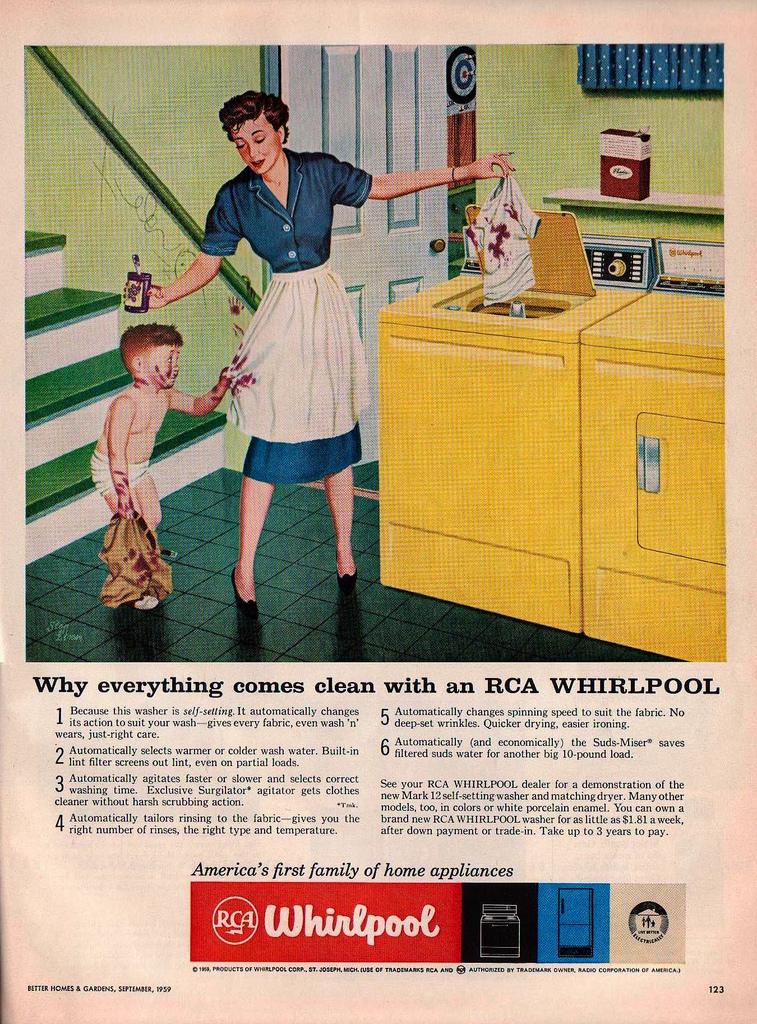This image is an antique advertisement for Whirlpool washer and dryers from Better Homes and Gardens, dated September 1959, appearing on page 123. It features a detailed illustration of a woman in a blue knee-length denim dress, high heels, and a white apron with her sleeves rolled up. She stands in a kitchen with a green tile floor and green stairs with white borders, putting a little boy's jam-stained shirt into a gold-colored washing machine. The boy, covered in jam, is handing over more dirty clothes while in his underwear, having already removed his pants. A dryer is partially visible next to the washer, with a box of detergent placed on a shelf above. The background has a vintage, yellowy-grayish tint, adding to the old-time feel of the scene. At the bottom, the Whirlpool logo is displayed on a red background beside a list of reasons why "everything comes clean with RCA Whirlpool," along with the tagline "America's first family of home appliances."